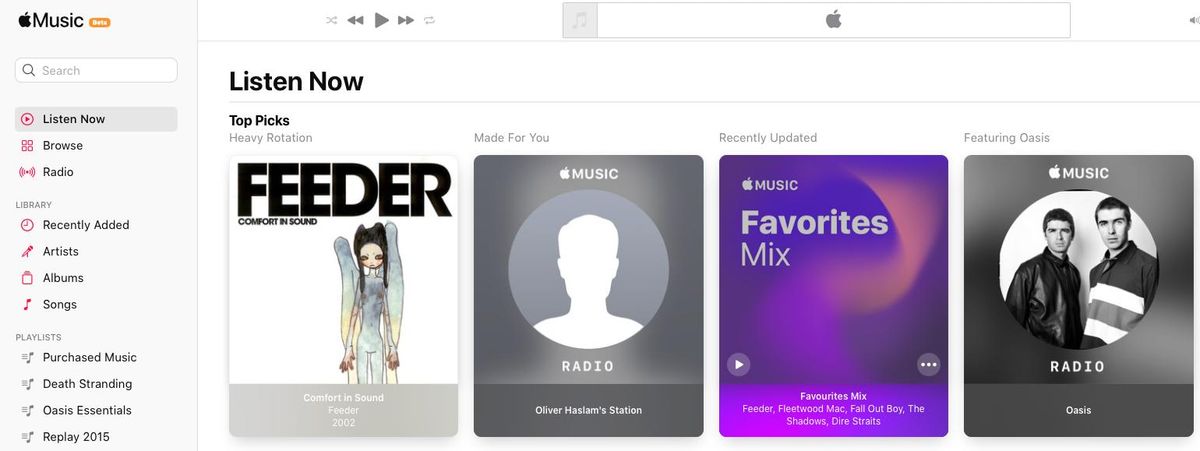In this image, we see the iTunes interface prominently displayed. In the top left corner, there are tabs for Music and Apple Music, with a 'Beta' label next to it. Directly below these tabs is a search field. Underneath the search field, various categories are listed, including "Listen Now," "Browse," and "Radio."

Moving further down the left side, we enter the Library section, which showcases options like "Recently Added," "Artists," "Albums," "Songs," "Playlists," and "Purchased." Specific playlists and music collections are visible within the Library, such as "Death Stranding," "Oasis Essentials," and "Replay 2015."

In the main content area, several sections are featured, including "Listen Now," "Top Picks," and "Heavy Rotation." Individual music selections such as Feeder's "Comfort in Sound," favorite mixes, and stations like the Oliver Haslam Station are displayed. Notable artists and bands, including Fleetwood Mac, Fall Out Boy, The Shadows, and Dire Straits, are also highlighted.

At the top of the page, playback controls are clearly visible, including buttons for Previous, Next, Play, Shuffle, and Repeat.

The interface integrates various elements from Apple Music, Radio, and personal music collections, making it a comprehensive hub for all music-related activities.